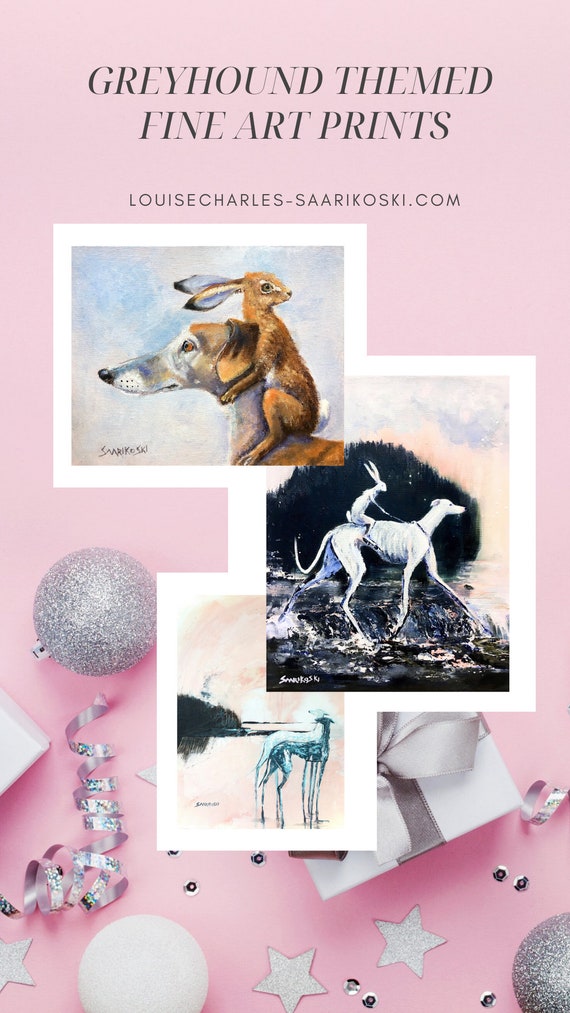The advertisement is set against a pink-purple background embellished with grey glittery stars, silver sequins, and golden and white Christmas balls, along with twisted silver ribbon adding a festive touch. At the top, in bold black capital letters, the text reads "Greyhound themed fine art prints," followed by the artist's website, louisecharles-saarikoski.com. The main body of the ad showcases hand-drawn illustrations of Greyhounds. There are four small images: one features a dog with a bunny clinging to its neck, another shows a bunny sitting on a Greyhound's back, and a third depicts a white dog standing with part of the image obscured by an overlapping picture. The artwork emphasizes the serene and detailed depiction of the Greyhounds accompanied by playful rabbits.